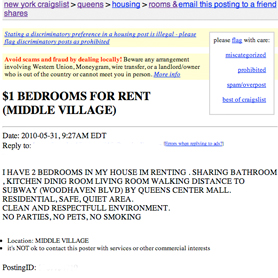**Caption:**

A nostalgic glimpse into a late 90s-style web interface, possibly originating from an old Craigslist page. The image is small, making the text blurry when zoomed in. The page features a primarily white background with purple and blue text indicative of previously clicked links and various colored texts for different sections of the page.

At the top, purple text represents clicked links such as "Rooms" while blue text includes "New York," "Craigslist," "Queens," and "housing." In this cluttered layout, a yellow banner with underlined blue text warns against discriminatory preferences in housing posts, advising users to tag such content as prohibited.

Below, in another yellow rectangle, red text cautions users to avoid scams and fraud by dealing locally, emphasizing wariness of arrangements involving Western Union, MoneyGram, Wire Transfer, or absentee landlords. Accompanied by black text detailing specific scam warnings, a blue link offers more information.

To the right, a rectangular sidebar contains a mix of black and blue text including links such as "Please flag with care," "miscategorized," "prohibited," "sports," "overpriced," "spam," and "Best of Craigslist," all in blue and clickable.

The left section highlights a housing listing: "Bedrooms for Rent in Middle Village" in black text, dated "2010-05-31 7:27 AM EDT." The poster details their offer in all caps, mentioning two available bedrooms in a house, shared common spaces like bathroom, kitchen, dining room, and living room. The location is praised for its proximity to the subway and Queens Centre Mall, along with being a safe, clean, and respectful environment with restrictions on parties, pets, and smoking.

Lastly, bullet points summarize the location as Middle Village and note that contacting the poster for services or commercial interests is not permitted. Some text at the end remains too blurry to discern.